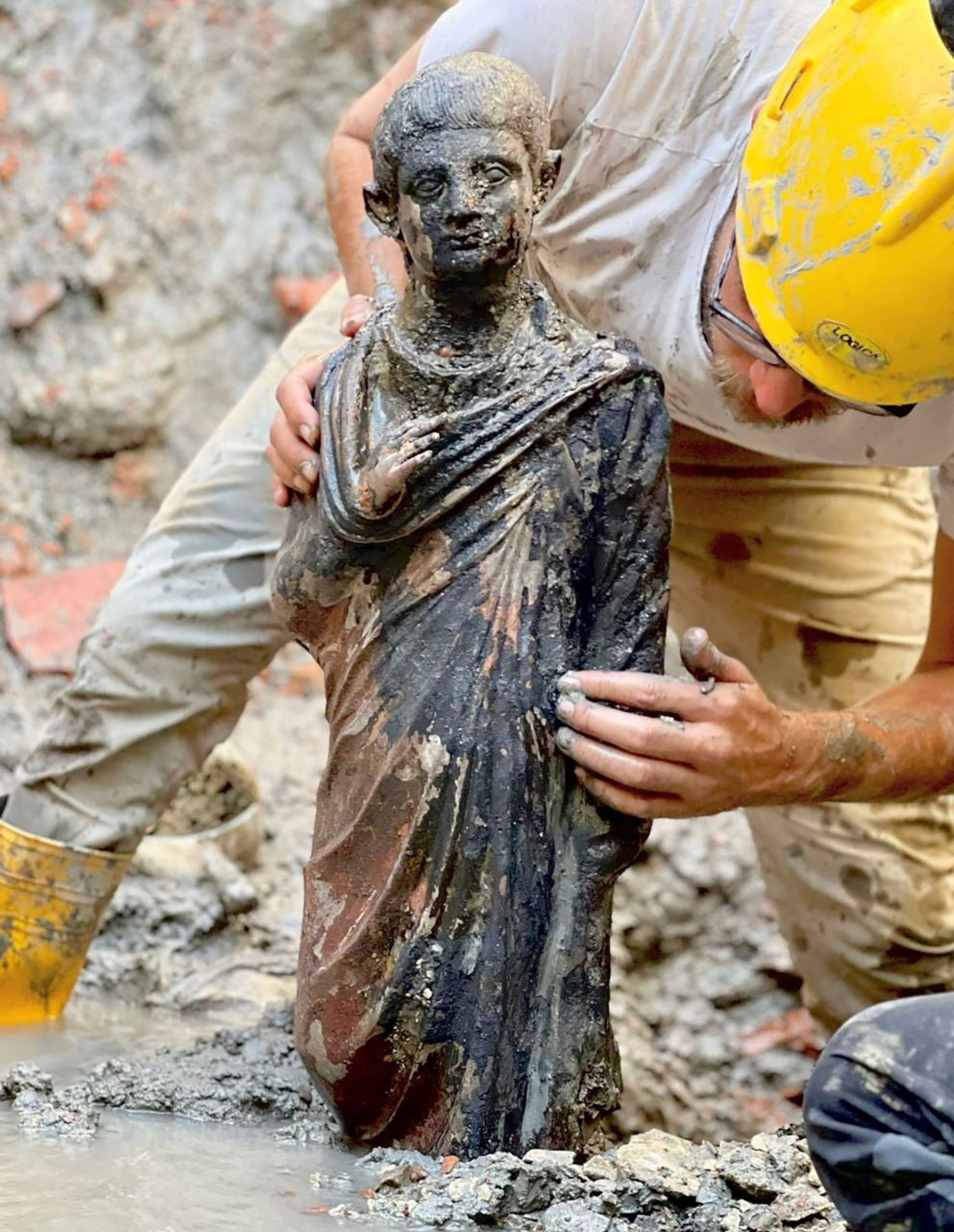In the image, a man, possibly an archaeologist, is carefully holding and examining a newly unearthed statue. The statue, which appears aged and weathered, features a man in a loose-fitting robe with one hand down by his side and the other hand crossing his chest as if held by a sling. The statue's colors include black, white, brown, rust, and beige, and it has short hair and a clean-shaven face.

The man studying the statue is standing in a muddy, watery area, perhaps indicative of a recent excavation site. He is dressed in a white t-shirt, dirty khakis, yellow rubber boots, a red construction helmet, and glasses with a mustache and beard. His expression is one of deep interest and care as he examines the statue, possibly ensuring it has suffered no damage. The scene suggests an important, possibly ancient find, pulling interest due to the statue's religious semblance and the meticulous efforts of its recovery. The tiny text on the helmet is unreadable, adding to the intrigue of the scene.